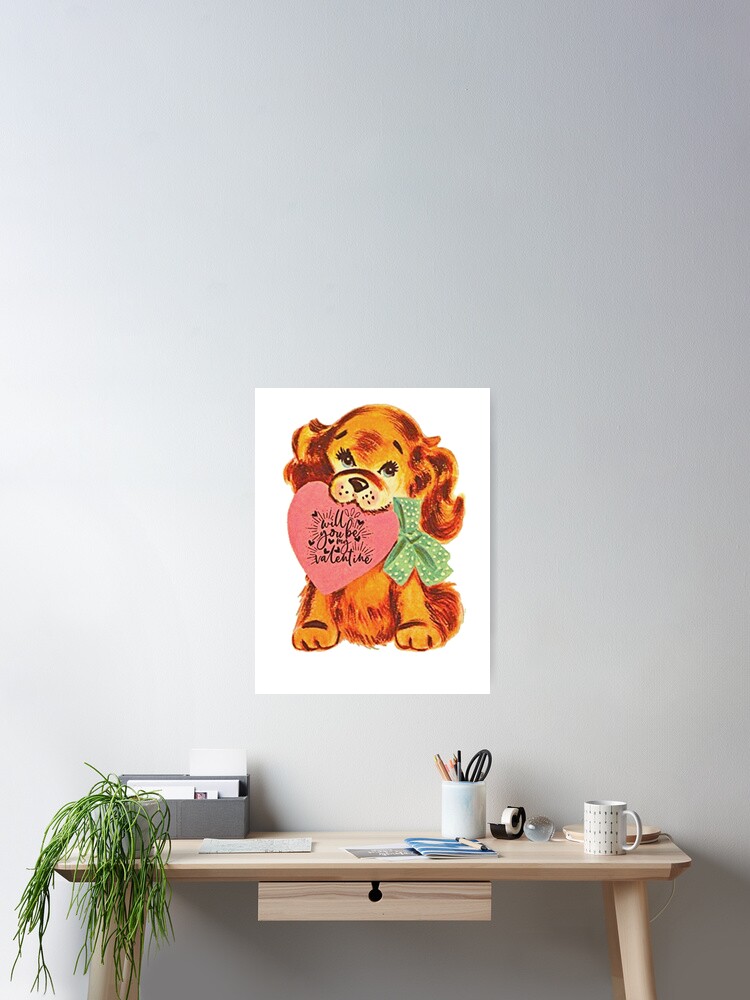The photograph depicts a light brown, blond wood desk with angled legs against a white wall. Centered along the desk is a small drawer with a keyhole-shaped cut-out. On the left side of the desk, a dark green, drooping plant reminiscent of a weeping willow sits in a short, gray vase beside a dark gray letter organizer filled with white papers. There is also a newspaper nearby. In the center of the desk lies an open magazine. To its right, a white ceramic cup holds a pair of black scissors and several pencils. Adjacent to the cup is a black tape dispenser, and next to that, there's a clear yet frosted circular object. Further to the right is a slender metal desk lamp with a cone-shaped shade. At the far right end of the desk, a beige-patterned coffee cup with a half-heart-shaped handle sits. 

Above the desk, a vintage valentine poster features a golden-colored puppy with long curly ears and blue eyes. The dog's fur showcases orange, burnt orange, and brown hues, with a beige snout and dark orange-brown accents. The puppy holds a pink heart with the black cursive message "Will you be my valentine?" in its mouth, and it wears a green bow with white polka dots around its neck.